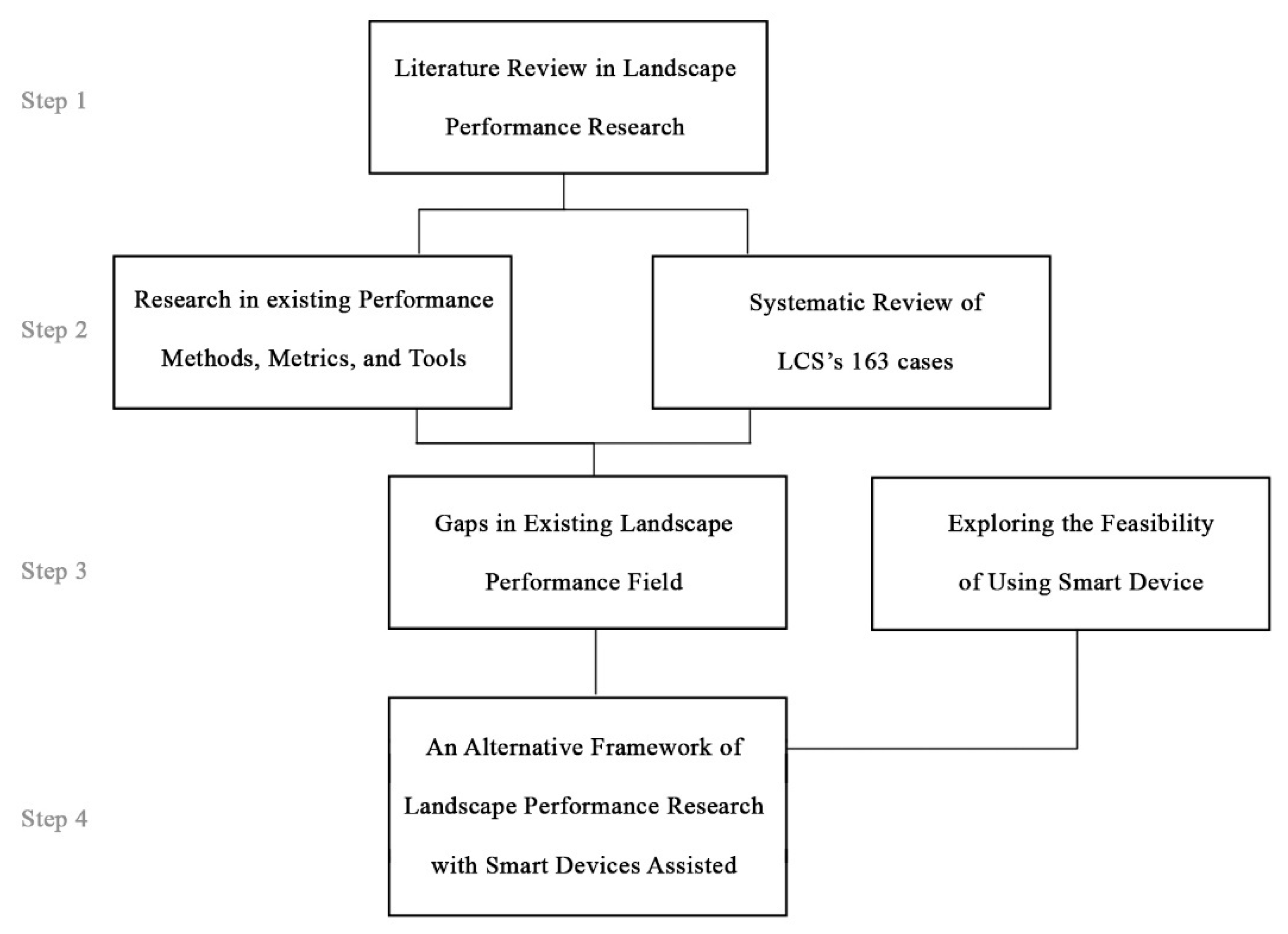The image presents a detailed four-step flowchart diagram for a research project. Along the left side, in light gray text, it lists vertically steps from 1 to 4. At the top, aligned with Step 1, there's a black-bordered white rectangle labeled "Literature Review and Landscape Performance Research." A line from this rectangle splits into two pathways leading to Step 2, which features two rectangles: the left one marked "Research and Existing Performance Methods, Metrics, and Tools," and the right one labeled "Systematic Review of LCS's 163 Cases." These two boxes converge into one rectangle at Step 3, titled "Gaps in Existing Landscape Performance Field." Adjacent to this is another box labeled "Exploring the Feasibility of Using Smart Devices." Finally, all pathways culminate at Step 4 with a rectangle stating "An Alternative Framework of Landscape Performance Research with Smart Devices Assisted."